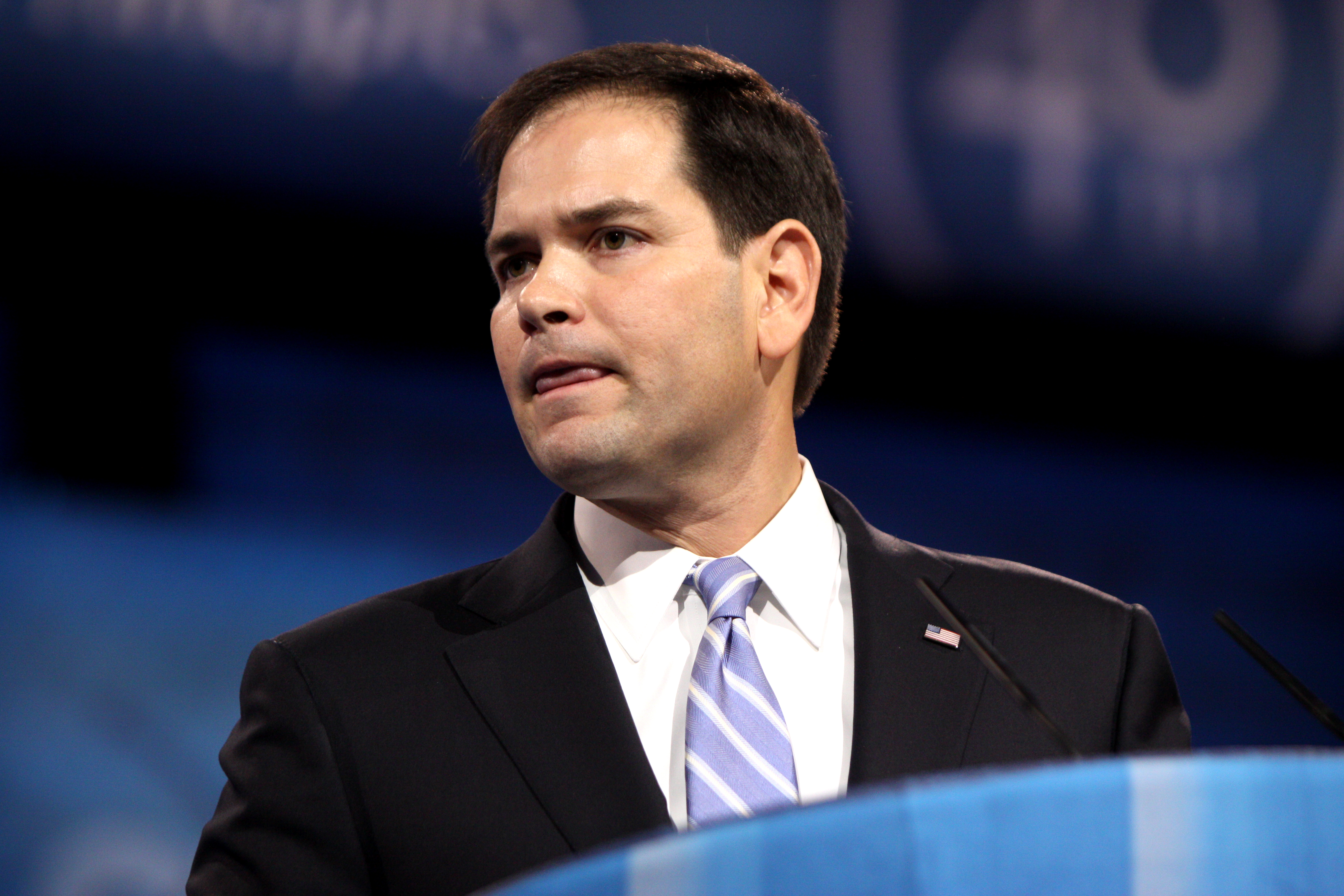The photo depicts a white man indoors, dressed in a grey suit, white button-down shirt, and a light blue and white striped tie, accessorized with an American flag pin on his left lapel. He has short brown hair with sideburns that reach the top of his ears, and he is looking slightly to the left with his tongue visible and his mouth slightly open. The image is cropped to show him from the head to chest level, with his arms resting at his sides. He seems to be standing at a podium, possibly made of glass, indicated by a blue reflection near the bottom of his jacket. The background features a blue band, a white band, and some unreadable white lettering, possibly including the number 40 inside a circle and a diagonal black stripe. The blurred elements suggest he might be on a stage, possibly addressing an audience or listening to a question. Two black objects, perhaps microphones, are visible on the podium in front of him.